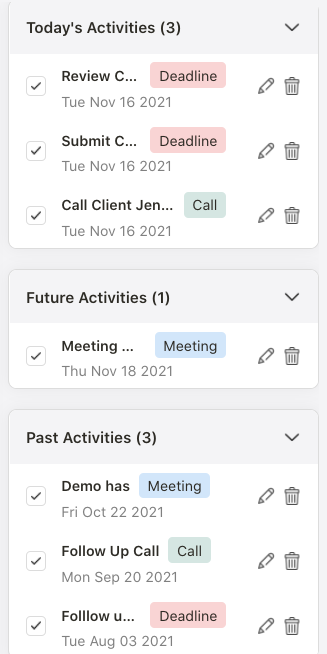Here we see a detailed screenshot of a mobile application interface used to manage various activities and tasks. The interface displays a drop-down screen titled "Today's Activities," which has been expanded to show three tasks for the day. The tasks are as follows:

1. **Review C** - The task has a deadline set for Tuesday, November 16th, 2021. It includes options to edit or delete it, represented by a pencil icon and a trash can icon, respectively.
2. **Submit C** - This task also shares the Tuesday, November 16th, 2021 deadline, marked with a notable pink deadline button. Similar to the previous task, it features options to edit or delete it.
3. **Call Client Gen** - Scheduled for the same date, this task includes a direct call button that allows the user to call the client without dialing the number manually. It also includes edit and delete options.

The interface further provides a section for "Future Activities," highlighting an upcoming meeting set for November 18th, 2021, with options to edit or delete it.

Lastly, the screen features a review of past activities:
- On October 22nd, 2021, there was a demo meeting.
- A follow-up call was made on September 20th, 2021.
- In August, an activity labeled simply "Follow" is listed.

All activities, regardless of their timeline, come with options to edit or delete. This comprehensive task manager offers a clear overview of ongoing, upcoming, and past engagements, likely designed for interaction with specific clients.